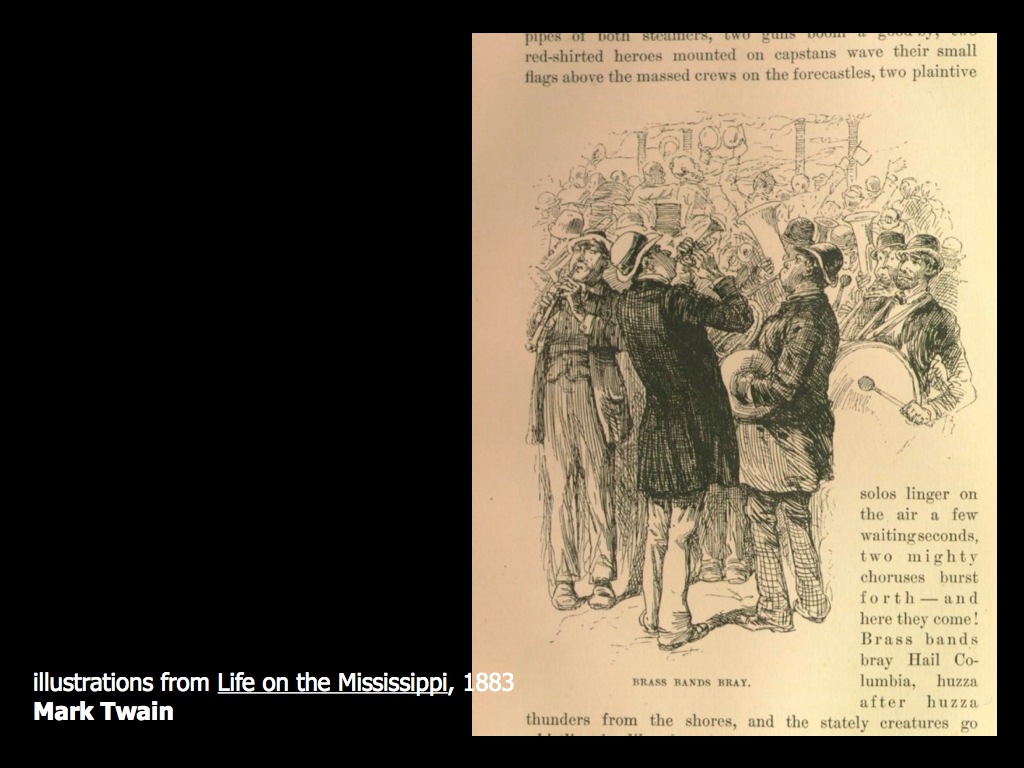This is an excerpt from the 1883 novel "Life on the Mississippi" by Mark Twain, featuring a detailed hand-drawn illustration on cream-colored paper. The illustration, likely done in pencil, is the focal point of the page. There's a caption beneath the drawing that reads "Brass Bands Bray." The image depicts a lively scene of men in leisure suits and bowler hats, playing various instruments, including tubas, drums, trumpets, cymbals, and possibly a trombone or flute. In the background, a crowd of cheering people is sketched in lighter, more indistinct lines, giving emphasis to the four musicians at the center. The page includes text above and below the illustration, with the visible portion of the book's text detailing a vibrant and energetic description of the bustling activity. The left side of the image displays white text against a black background, stating "Illustrations from Life on the Mississippi, 1883, Mark Twain," providing context for the origin of the illustration.